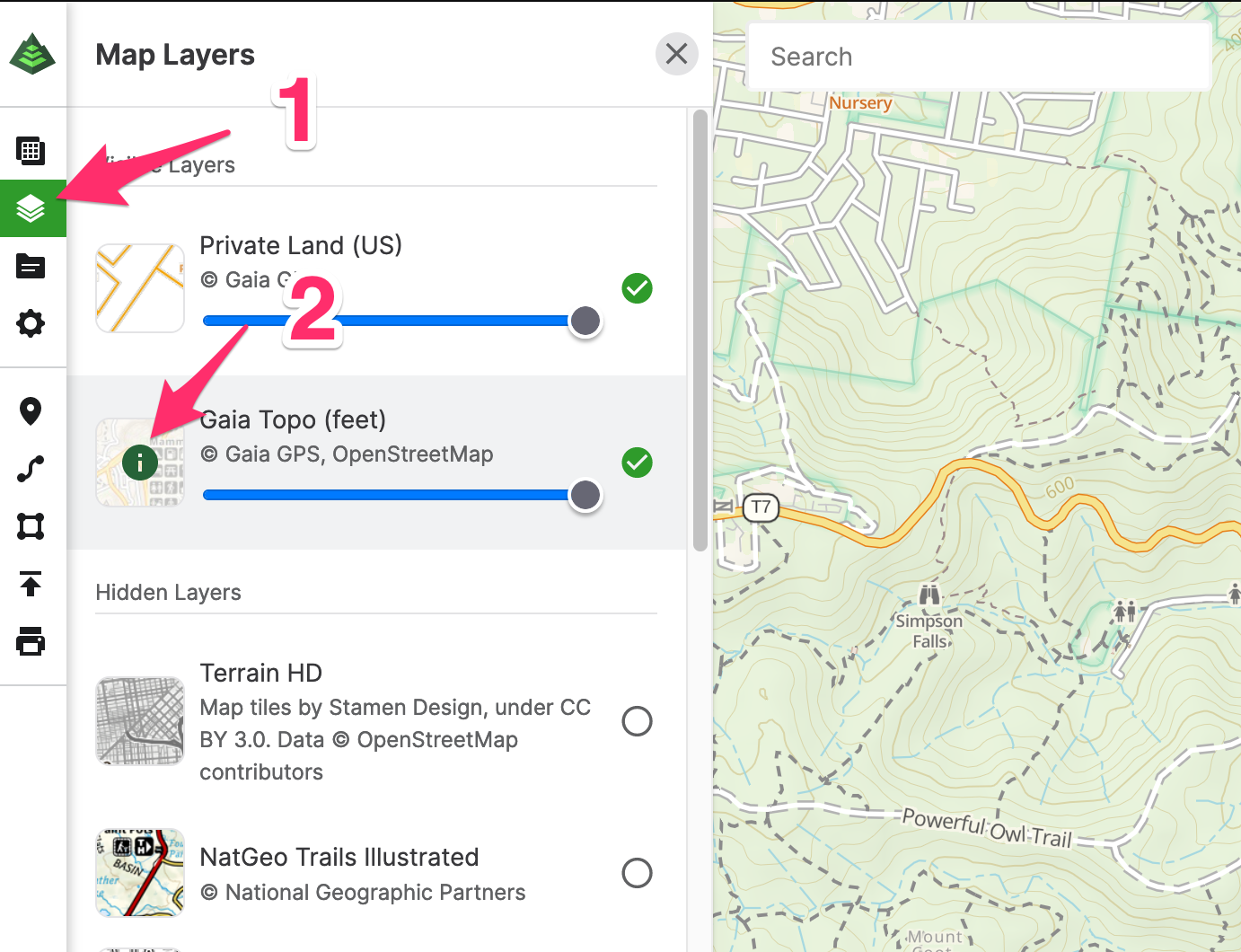The interface page is divided into two primary sections. On the left side, there is a column featuring a series of icons. At the top of this column, there is a green icon followed by text that reads "Map Layers." To the right of this label, a small "X" icon indicates the option to close this section. 

On the right side of the page, a detailed, green-tinted map is displayed, showing a network of unnamed roads. Towards the top of the map, a white search box is situated, containing the word "Search" in gray text, suggesting that users can type their queries here.

Among the icons in the left column, the third one from the top is highlighted with a green box around it. Adjacent to this, a small arrow points to the highlighted icon and is labeled with the number "1." Just below this highlighted icon, another section titled "Gaia Topo" appears. An arrow labeled with the number "2" points towards this section, directing attention to it. This detailed interface seems designed to help users interact with and customize their map layers effectively.